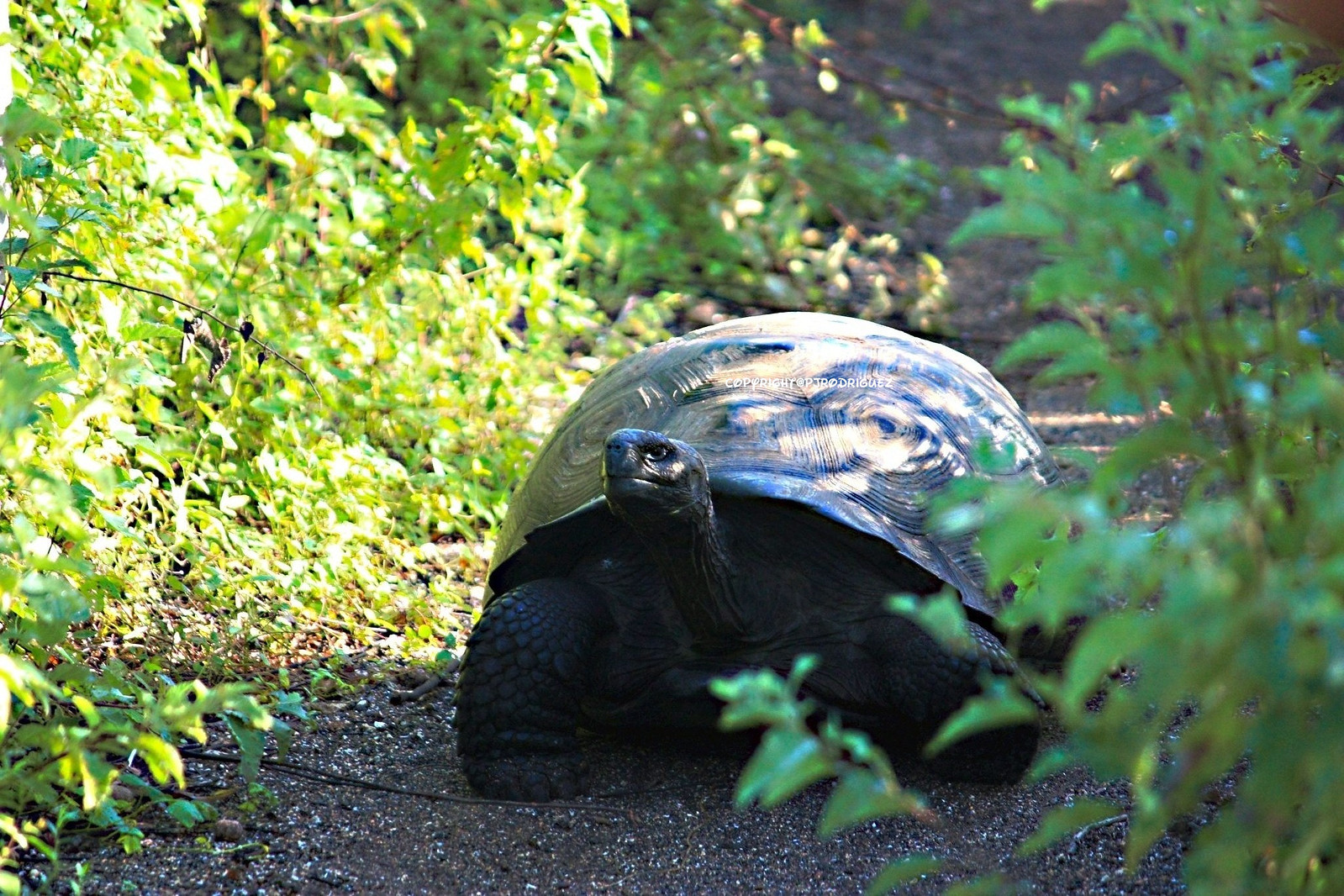A fairly large tortoise is walking towards us down a narrow gravel path, illuminated by daytime sunlight. The tortoise has a greenish-gray to dark gray complexion covering its head, legs, and neck, with visible scales on its front legs. Its dome-shaped shell is lighter brown, dappled with sunlight and casting shadows due to surrounding leaves. Small, faint copyright text is barely visible on its shell. The path is bordered by small plants, shrubberies, and dense greenery on both sides. The background features more of the dirt path, sparse vegetation, and a small hill, indicating the trail the tortoise likely took.